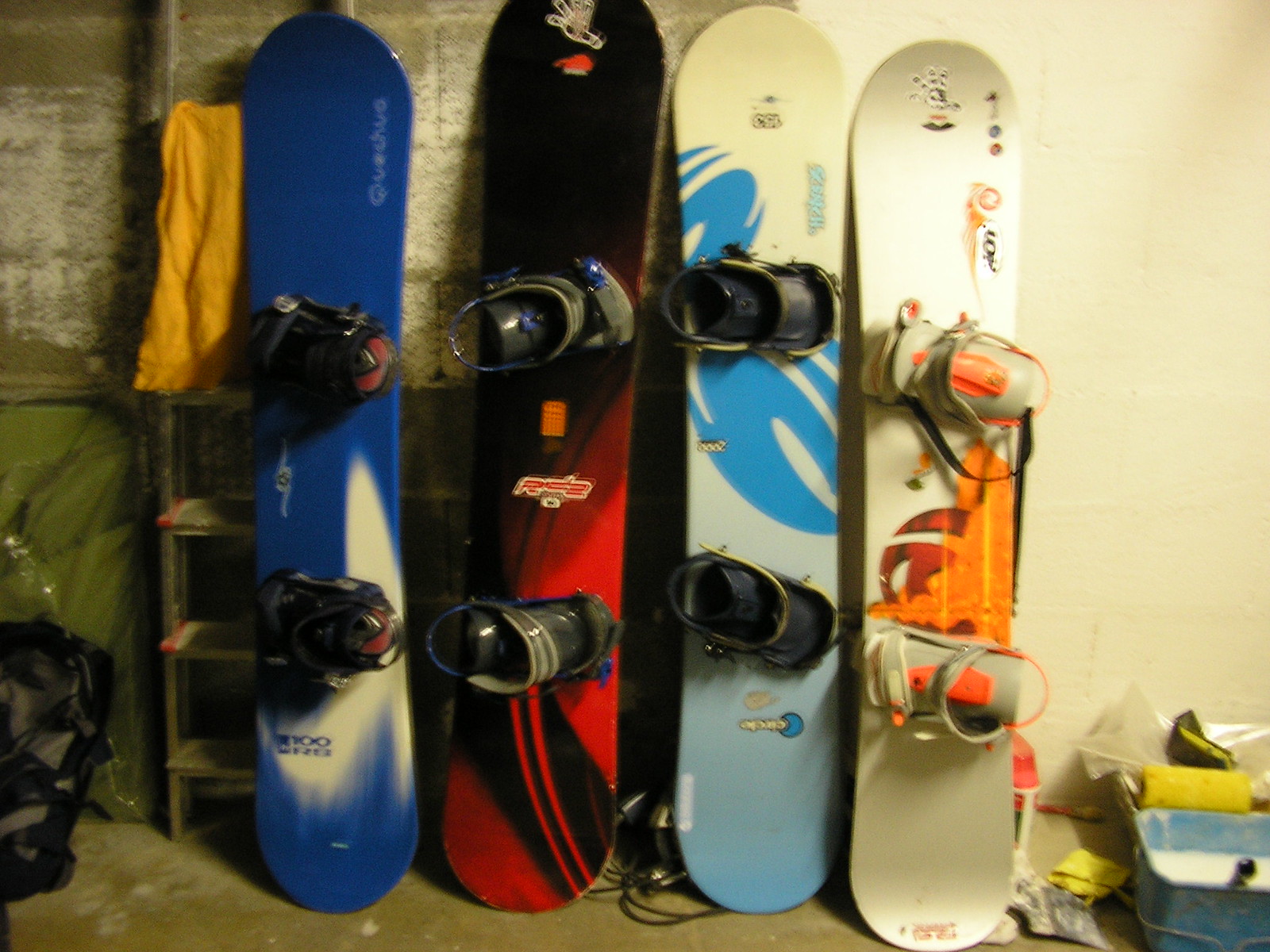This slightly blurred color photograph depicts four snowboards leaning vertically against a wall, presumably in a basement with concrete floors and unfinished brick and painted walls. From left to right, the snowboards feature distinct designs: the first is royal blue with a white pattern, the second is a striking black with a dark red design, the third sports a white and light blue background with swirly blue accents, and the fourth is predominantly white with an orange motif. Each snowboard has boot straps affixed at the center. Behind them, a ladder is visible, with an orange towel draped over it, positioned near the blue snowboard. In the lower right corner of the image, there is miscellaneous debris, including a bucket filled with a white liquid and squeegee yellow rollers. The scene suggests either an auction listing or a personal sale setup, capturing the snowboards in a casual indoor setting.